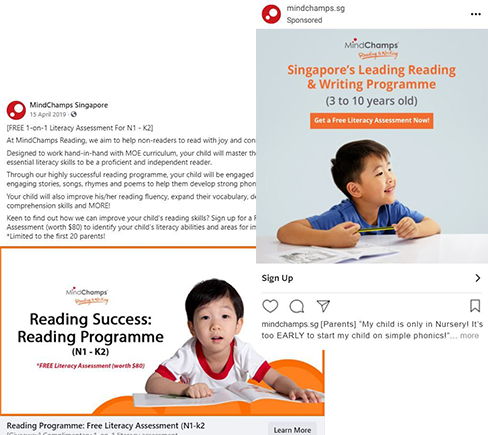### Detailed Caption:

This image presents two overlapping advertisements from Mindchamps.sg, prominently featured as sponsored content. The top photo is an Instagram post showcasing a promotional ad with the heading, "Singapore's Leading Reading and Writing Program" catering to children aged 3-10 years old. At the top, "Mindchamps.sg Sponsored" is clearly visible. Centrally, the Mindchamps logo is displayed, conveying brand identity. In the image, a young Asian boy dressed in a blue shirt sits at a white table, holding a pencil and engaging with a workbook. Below this visual, there's a bold, orange rectangular button with the call-to-action text, "Get a free literacy assessment now," written in white font. The caption below this post reads, "Mindchamps.sg Parents: My child is only in nursery. It's too early to start my child on Semblance Funds..." followed by an option to see more.

The second photo, partially obscured beneath the first, features another ad from Mindchamps Singapore dated 15 April 2019. It is marked as a public post. The key message highlights a free one-on-one literacy assessment for children in N1 through K2. The text outlines how Mindchamps Reading aims to help non-readers develop a love for reading. Emphasizing alignment with the MOE curriculum, it assures that children will gain essential literacy skills, engage in stories, songs, rhymes, and poems, and improve their phonics, reading fluency, vocabulary, and comprehension. The ad pursues enlisting parents by offering a free reading assessment valued at $80, available to the first 20 participants. Below, within an orange rectangular outline, there is an image of another young Asian boy in a white and red shirt leaning over a workbook. To the left of this picture, it reads "Reading success, Reading program (N1 through K2)," with a reminder of the free literacy assessment worth $80 at the bottom right. The post concludes with a "Learn more" option, encouraging further engagement.

The Instagram interface elements, such as the heart, comment, share, and bookmark buttons, along with engagement options such as signing up, are clearly visible, underscoring the promotional nature of these overlapping visuals.